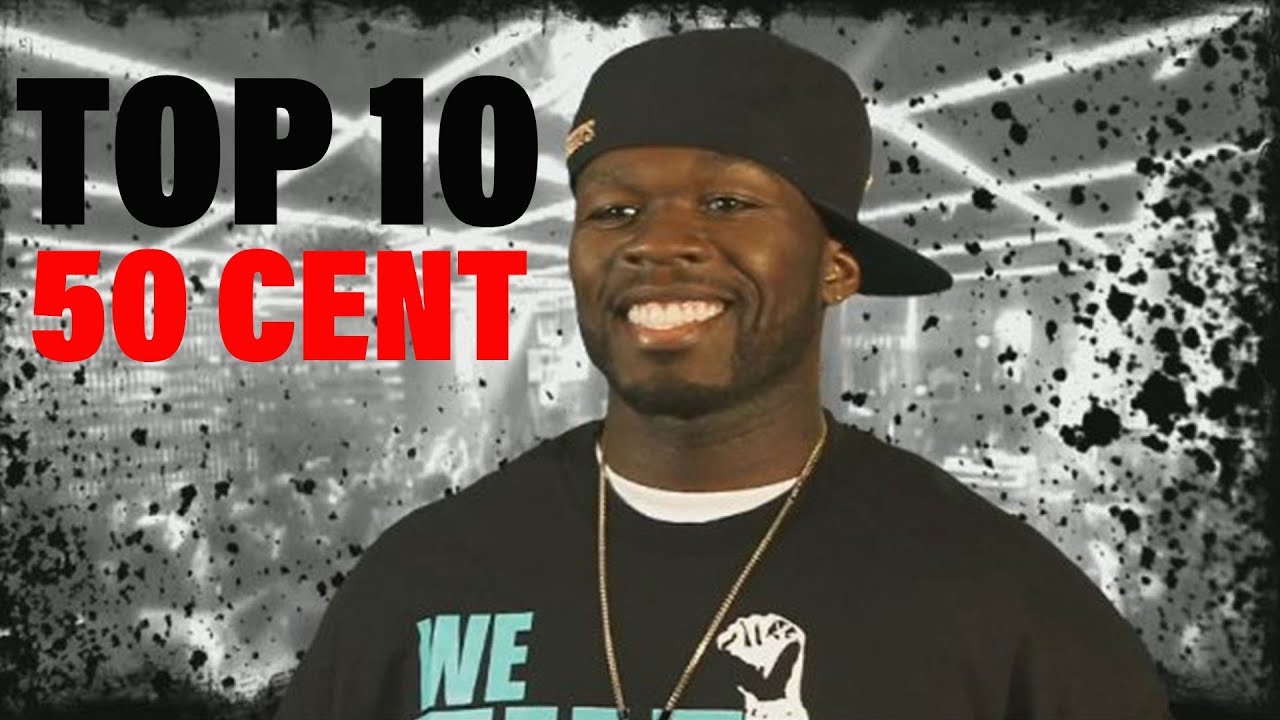The image is a color photograph of the rapper 50 Cent, who is a smiling Black man looking to the left side of the frame. He wears a black baseball cap turned backward, revealing his short stubble and meticulously groomed mustache and beard. 50 Cent is dressed in a black graphic T-shirt layered over a white undershirt, complemented by a gold chain around his neck. The T-shirt has the word "WE" visible at the top. In the background, there is a black-and-white photo that gives the impression of a club scene, dotted with black spots or "blushes." Overlaying the image, in the top left corner, are the words "Top Ten" in black letters and "50 Cent" in red letters.